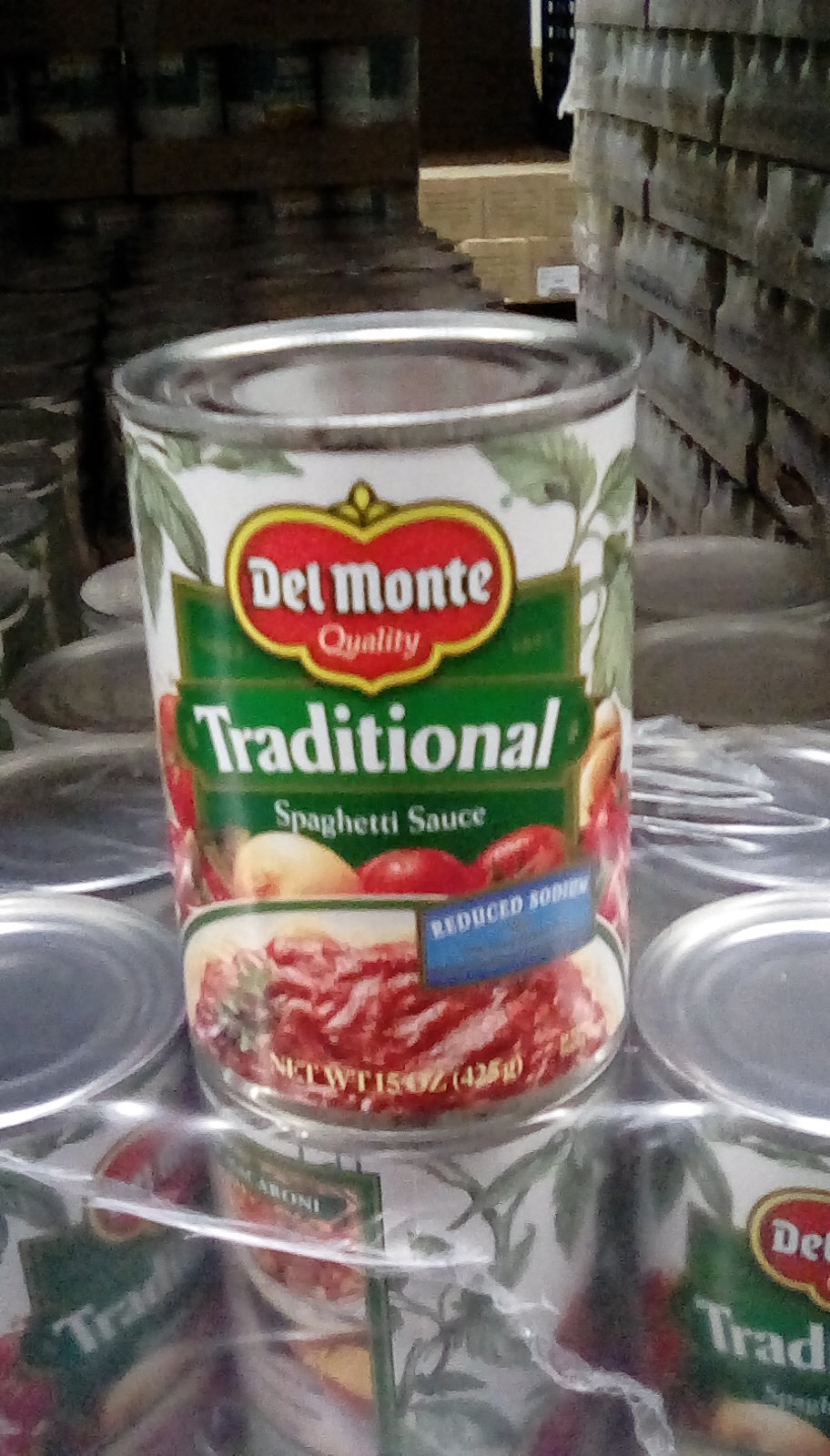In a dimly lit storage area of a grocery store or warehouse, a photo captured on a cell phone showcases a 425-gram can of Del Monte Traditional Spaghetti Sauce. The can stands out against a backdrop of shrink-wrapped cases of various products, with some distant boxes faintly illuminated. The can itself features a predominantly white background adorned with green leaves, likely representing the herbs in the sauce. Central to the design is the distinctive Del Monte logo, characterized by its unique shape, red background, and white font. Beneath the logo, a green banner displays the word "Traditional" in white text, followed by "spaghetti sauce" in the same font. The lower section of the label depicts ripe tomatoes and onions, accompanied by a bowl of the rich, red pasta sauce. The bowl also bears a small, blue label with white text indicating "reduced sodium." This detailed packaging evokes the classic and wholesome nature of Del Monte's spaghetti sauce.